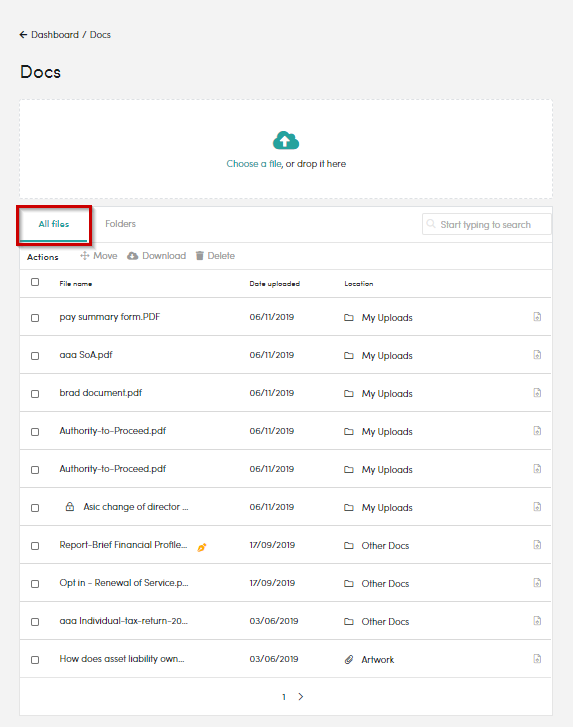**Screenshot of Document Management Dashboard**  

The image is a screenshot showcasing a document management program or dashboard. At the top, it displays the navigation options with labels such as "Docs," "Options," and "Dashboard" highlighted as "Dashboard/Docs." 

The primary section features a prominent upload area distinguished by a large, dotted box with a cloud and an upload icon in the center. Inside the box, there is text instructing users to "Choose a file or drop it here."

Above the main content area, there are tabs for categorizing files. The highlighted tab, labeled "All Files," is indicated by a red box, while adjacent to it is another tab labeled "Folders."

Directly below these tabs, a search bar prompts users to "Start typing to search." Below the search bar, there are action buttons for moving, downloading, or deleting files.

The dashboard is organized into columns with headers for "Actions," "File Name," "Date Uploaded," and "Location." The list contains ten files, each with its details as follows:

1. **Pay Summary Form.pdf** – Uploaded on 06/11/2019
2. **ASOA.pdf** – Uploaded on 06/11/2019
3. **Brad Document.pdf** – Uploaded on 06/11/2019 – Located in "My Uploads"
4. **Authority to Proceed.pdf**
5. **Authority to Proceed.pdf**
6. **Sick Change of Director...**
7. **Report Brief Financial Profile...** – Classified under "Other Documents"
8. **Opt-in Renewal of Service.p...**
9. **Individual Tax Return 20...**
10. **Asset Liability Own...**

The layout is typical for an online document management system, where users can upload, manage, and search for files efficiently. The first page of the document list is depicted in this screenshot.